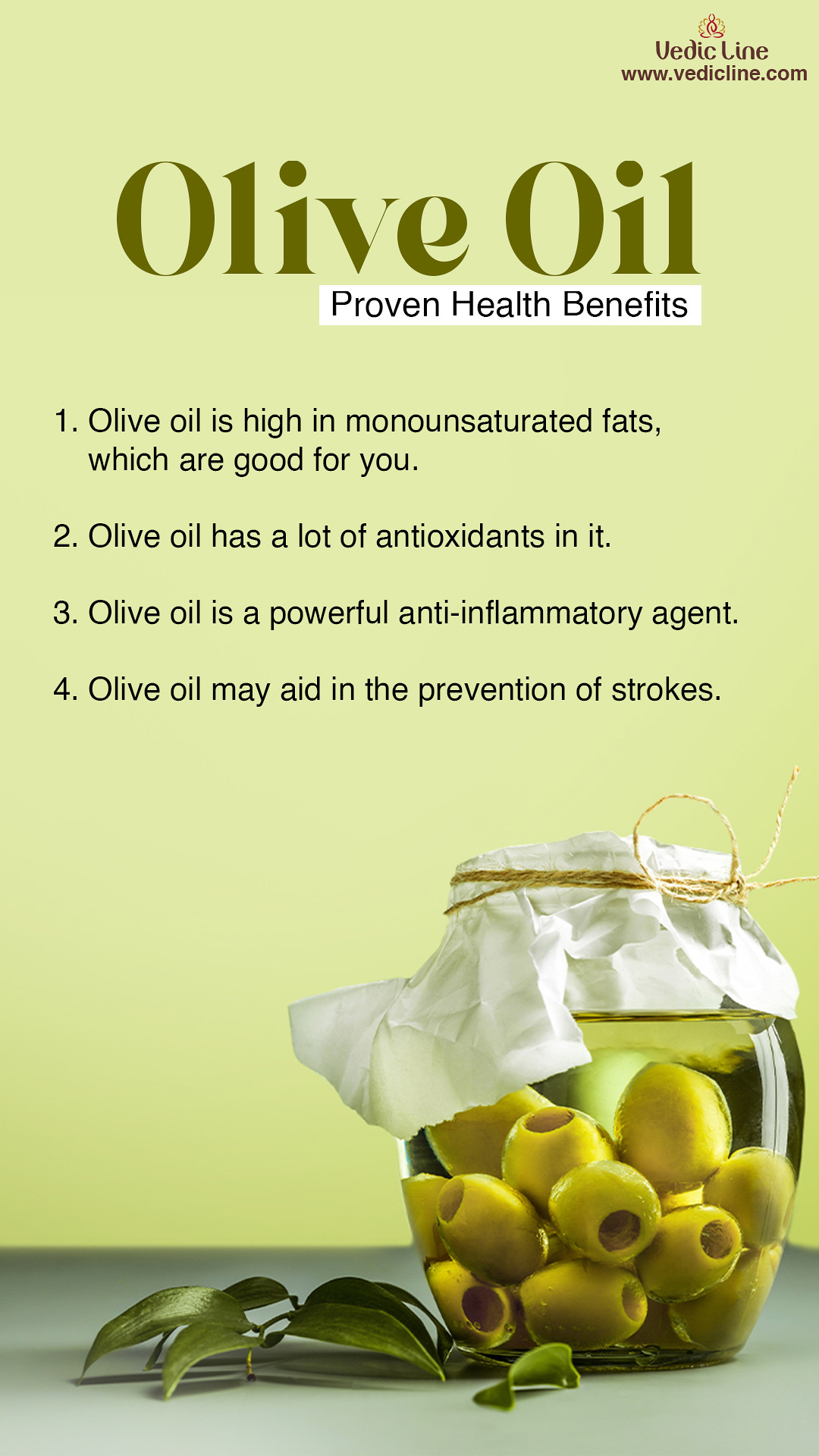The image presents information about the health benefits of olive oil against a gradient background that transitions from a light sage green at the top to a darker mint green at the bottom. Central to the image is a round, wide glass jar filled with green olives immersed in olive oil. The jar is adorned with a white cloth cover, secured with a brown twine string. To the left of the jar, green olive leaves are placed as an accent.

Text overlay on the image reads "Olive Oil" in a green olive color, followed by "Proven Health Benefits" in black text on a white background. Below this heading, four key health benefits of olive oil are listed:
1. Olive oil is high in monounsaturated fats, which are beneficial for health.
2. Olive oil contains a significant amount of antioxidants.
3. Olive oil is a powerful anti-inflammatory agent.
4. Olive oil may aid in the prevention of strokes.

Additionally, the text "Vedic Lyme, www.vediclyme.com" is present, reinforcing the source of the information. The light green background and light table enhance the overall olive-themed color palette, and the jar of olives casts subtle shadows, adding depth to the image.